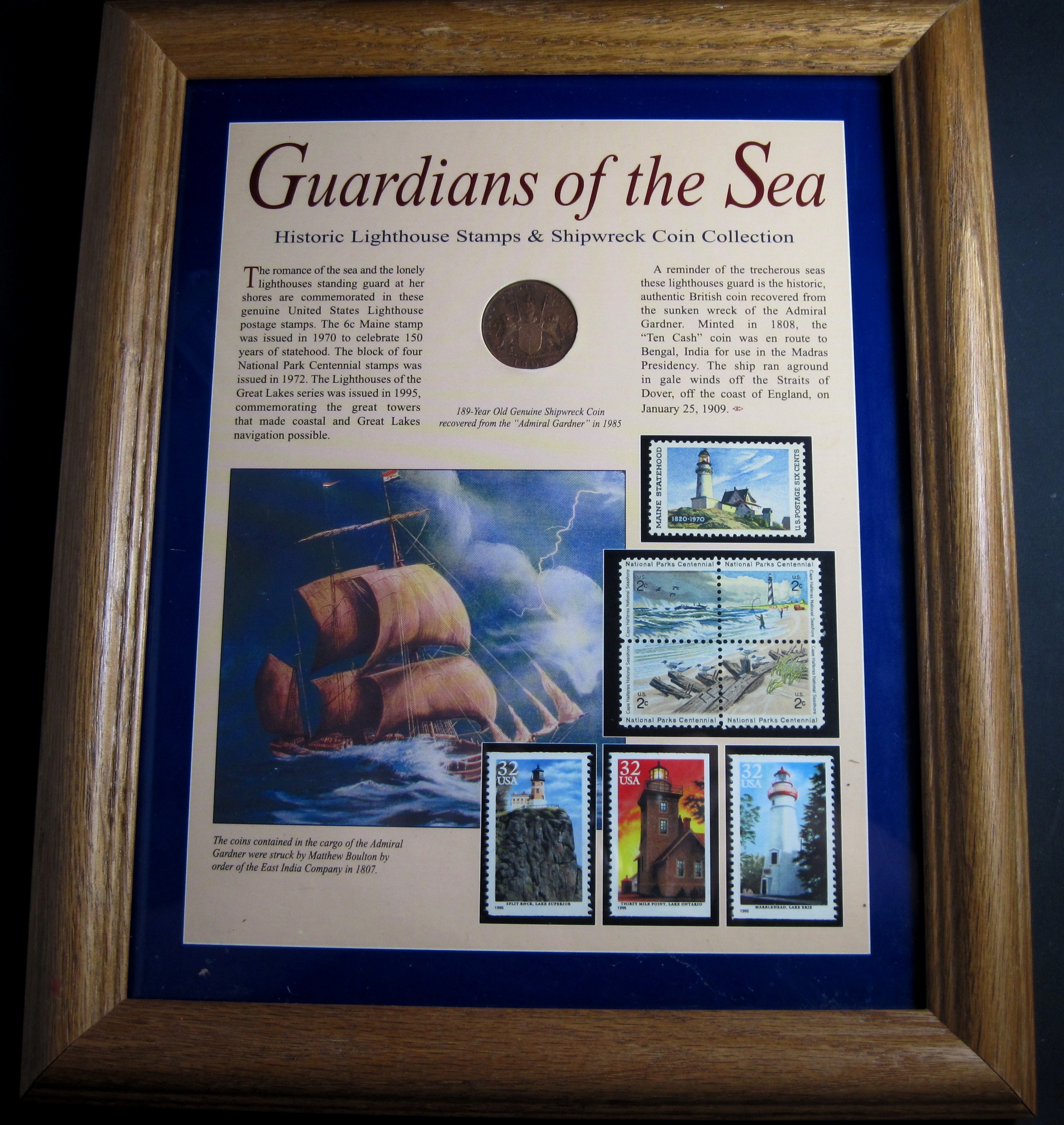This is a detailed color image of a framed display titled "Guardians of the Sea: Historic Lighthouse Stamps and Shipwreck Coin Collection." The display, enclosed in a wooden frame and mounted on a navy blue mat, features a white background with the title in red and blue text. The centerpiece is a paper with two columns of descriptive text and an array of historic lighthouse postage stamps, predominantly showcased in the lower right-hand corner. The stamps, including the six-cent main stamp from 1970, a block of four National Park Centennial stamps from 1972, and the Lighthouses of the Great Lakes series from 1995, celebrate iconic lighthouses vital to coastal and Great Lakes navigation. A poignant reminder of the hazardous seas is embedded within the display—a genuine British coin from the sunken wreck of the Admiral Gardner, minted in 1808 and intended for Bengal, India. This coin symbolizes the perils of maritime voyages, having been recovered from an 1809 shipwreck off the coast of England. The lower left of the display features a vivid painting of a ship battling a stormy sea, complete with dramatic clouds and lightning, adding a timeless visual narrative to the collected historical artifacts.